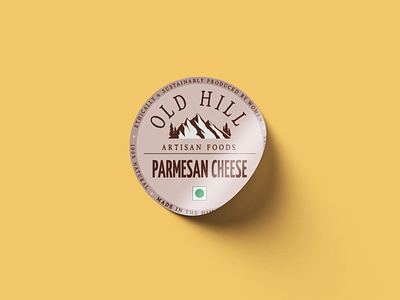This image features a small horizontal rectangular piece of yellow paper with a partially attached label. The top left corner of the label is adhered to the paper, while the right side is slightly lifted, suggesting the adhesive might be inadequate or it wasn't properly pressed down. The label itself is circular, with a background in a light pinkish hue and a dark purple border encircling it. 

At the top of the label, "Old Hill" is prominently displayed in dark maroon letters. Below this, there is a mountain symbol followed by the words "Artisan Cheese" in smaller text, accompanied by a horizontal line beneath it. The central part of the label features "Parmesan Cheese" in bold, dark maroon capital letters. At the bottom, a white square encloses a small green circle, perhaps the company’s logo. This descriptive label is stuck to a block of cheese intended for grating, commonly enjoyed by many despite the commentator’s personal taste preferences.